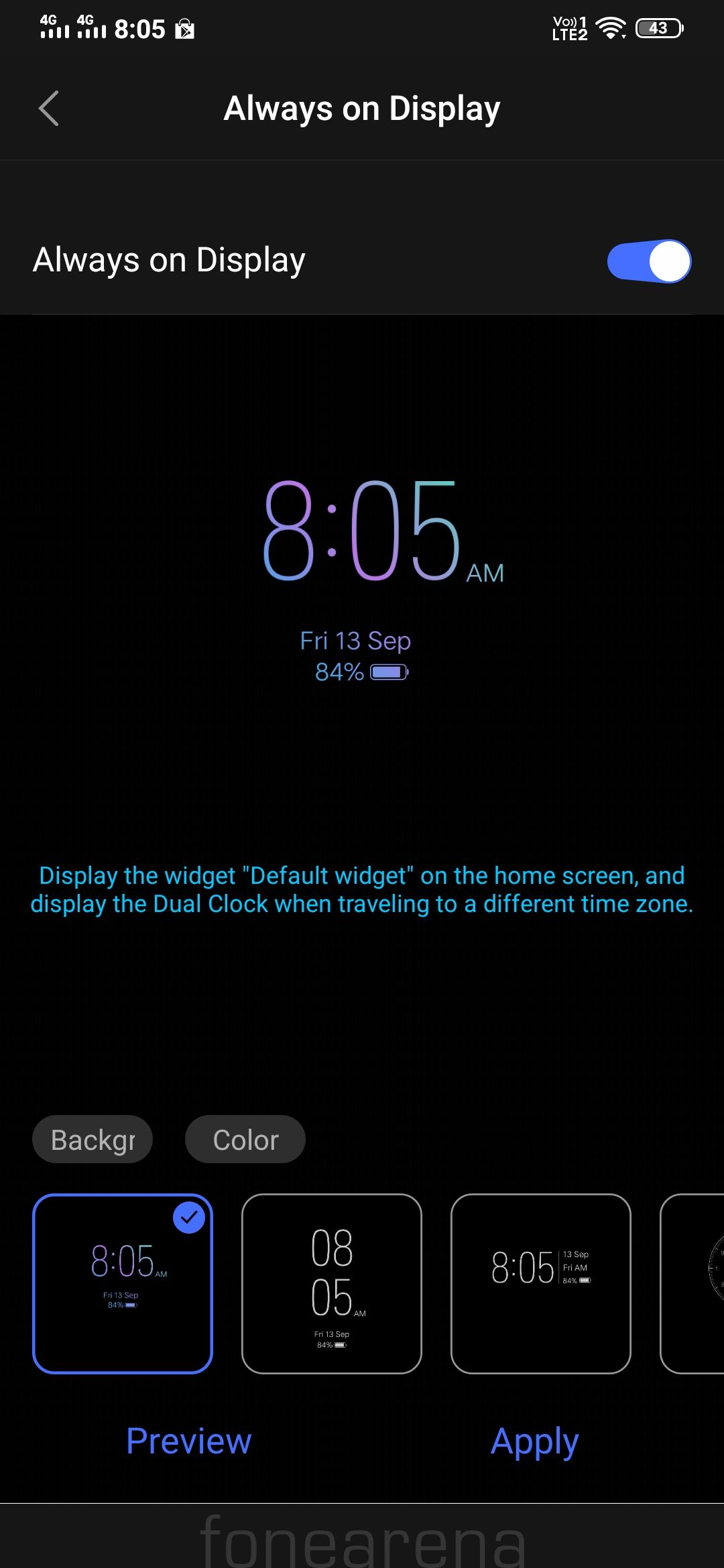This is a color image, appearing as a screenshot from a mobile phone's settings interface. The background is predominantly black, with white text and some elements highlighted in blue and multicolored text. 

In the upper-left corner, the status bar shows '805' alongside two 4G icons with four signal bars each, implying the presence of dual SIM cards. To the right, the status bar displays a Wi-Fi icon and a battery icon.

Centered below the status bar, white text reads "Always On Display," accompanied by a back arrow. Following that, on the left side, the text "Always On Display" is repeated with a blue slider next to it indicating that this function is enabled.

In the middle of the screen, the current time is displayed as 8:05 AM, outlined in a gradient of blue and purple hues. Directly below the time, the date is shown as "Friday, 12th September," and an 84% battery indicator is visible.

Further down, blue text instructs, "Display the default widget on the home screen and display the dual clock when traveling to a different time." There are white-text buttons for "Backlog" and "Color" on the left side.

At the bottom section of the screenshot, four square icons represent different clock styles to choose from. Three clocks are clearly visible, and part of a fourth can be seen. The first clock on the left is selected, denoted by a blue checkbox and a blue outline. The subsequent clock styles show the time as 8:05, with distinguishing text elements like "08" over "05" on the second clock, and additional text to the right of the time on the third clock.

Below these options, the text "Preview" appears in blue on the left, and "Apply" is on the right. A horizontal bar separates these options from the rest of the screen.

At the very bottom, a partial watermark is visible, indicating the image is sourced from the website PhoneArena.